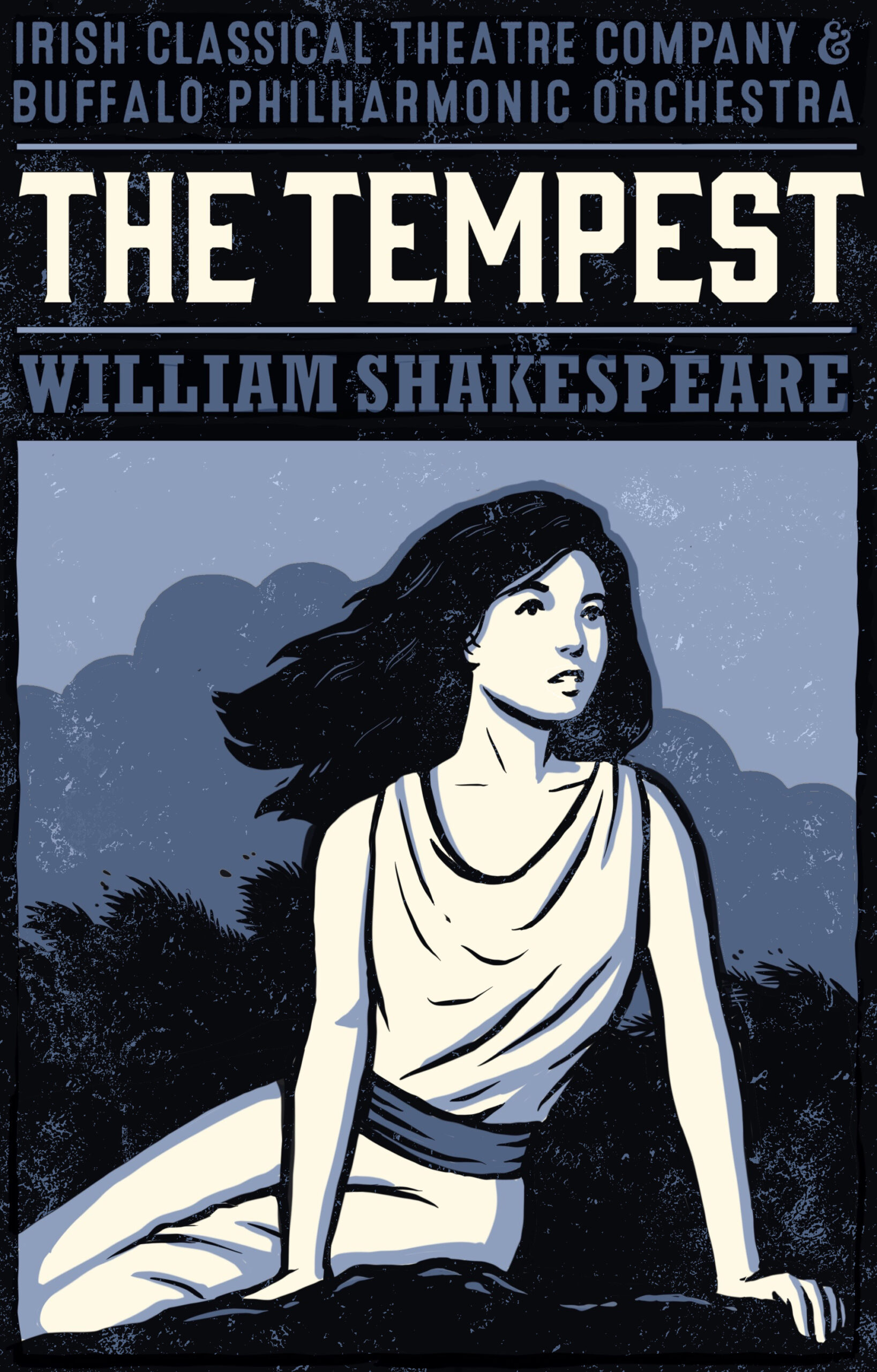A poster titled "The Tempest" by William Shakespeare, presented by the Irish Classical Theatre Company and the Buffalo Philharmonic Orchestra, depicts a detailed illustration of a woman in a classical style set against a mountainous, wooded background. The woman, portrayed in black and white with shades of blue and gray, has long black hair flowing in the wind. She is dressed in a white outfit with a blue belt and is seated on a rock, propped up by her arms, gazing into the distance with an anxious expression. The sky behind her ranges from light blue to dark, creating a dramatic and evocative setting for the play’s advertisement.